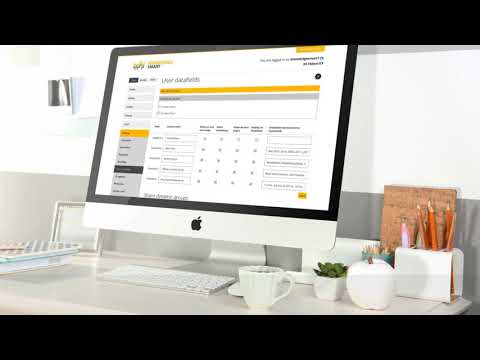This image depicts a meticulously organized and modern office desk setup, likely a stock photo. At the center of the gray desk stands an Apple iMac with a white stand, displaying a website that resembles a data sheet with labels, numbers, and yellow banners. The sleek white keyboard and mouse sit directly in front of the screen. To the right, a small white coffee cup, a green succulent in a white vase, and a white pencil holder add to the tidy arrangement. A distinctive white sculpture of an apple with a brown stem is also present, enhancing the minimalistic aesthetic. On the left side of the desk, there are neatly placed books and a notepad. The overall color scheme is dominated by white and gray tones, contributing to the clean, contemporary design of the workspace, which may even be 3D rendered due to its pristine appearance.